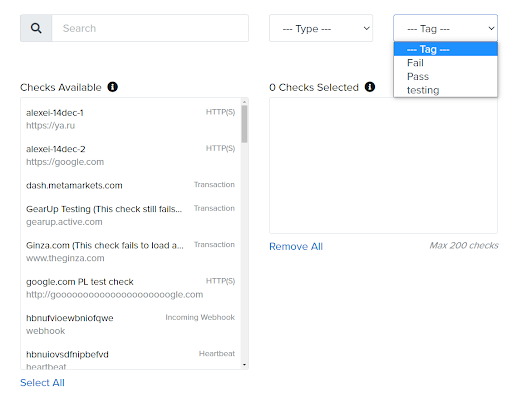The image depicts a web checker interface, designed for monitoring and evaluating multiple websites or services. At the very top left corner, there is a search bar accompanied by a magnifying glass icon. Adjacent to the search bar is a dropdown menu labeled "Type." On the extreme right side of this top section is another dropdown menu labeled "Tag," which, when clicked, reveals three options: "Fail," "Pass," and "Testing."

Beneath these top elements, the interface is divided into two side-by-side sections. The left section is titled "Checks Available," with a small black circular information button next to the title. This section contains a scrollable list of options, which include different websites, transactions, incoming webhooks, and heartbeats, although only these four are visible in the current view. There is a "Select All" option in blue located at the bottom of this list.

To the right of the "Checks Available" section, there is another box labeled "Zero Checks Selected," also accompanied by a black circular information button. This box is currently empty. Below this box is a blue "Remove All" button. Additionally, a note beneath the second box indicates a limit of "Max 200 checks."